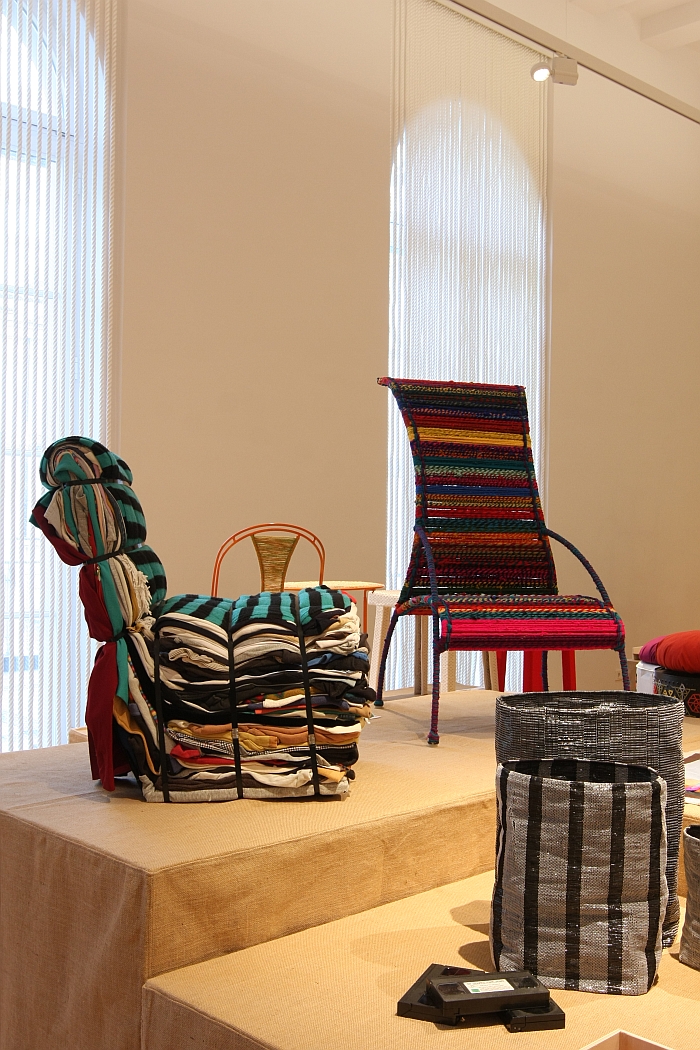This color photograph, taken inside a room that resembles a museum or exhibition space, showcases an eclectic furniture display against a backdrop of two domed windows with white blinds. In front of these windows, two wooden platforms covered in beige fabric hold a pair of unconventional, artistically rendered chairs. The left chair, resembling a pile of clothing bound with black straps, appears crafted from recycled materials. The right chair features a colorful woven pattern in shades of red, green, yellow, and blue, with black arms and legs. In the foreground, a lower platform displays two silver bins, one with vertical stripes, alongside three VHS tapes stacked on top of each other. The overall composition exudes an artistic and avant-garde ambiance, emphasizing the chairs' vivid, recycled materiality and unique design.